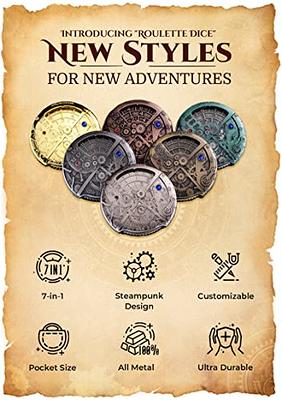This image is a vintage-style advertisement poster, resembling those from the 1500s with worn and beaten edges and a brownish paper color, indicating its old-fashioned aesthetic. At the top of the poster, bold text introduces "Roulette Dice: New Styles for New Adventures." The poster showcases six distinct circular-shaped metal dice, each exhibiting unique steampunk designs and vibrant colors. Key features highlighted include their 7-in-1 capability, steampunk design, customizability, pocket-sized convenience, all-metal construction, and ultra-durability. These attributes are described through various symbols around the image, enhancing the informational aspect. The poster's overall layout, including textual descriptions and detailed imaging, effectively captures the allure and innovative features of the Roulette Dice.